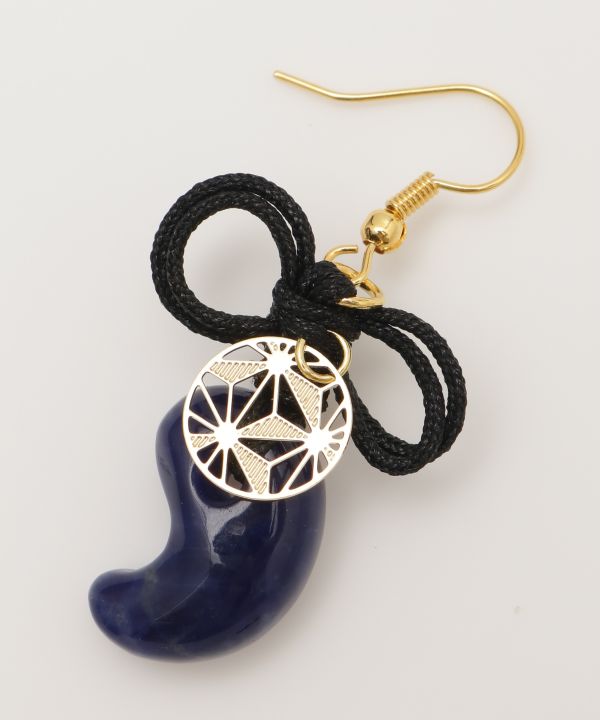This close-up image showcases a detailed earring with multiple intricate elements. The earring features a gold hook, typical for piercings, attached to a very thin black rope tied in a knot with two loops flanking the knot. A small gold circular ornament is entwined within the black rope. Below this, a more complex silver circular piece, adorned with an ornate design of interconnected lines and shapes, hangs from the rope. The design within the silver piece includes lines leading into smaller circles and rectangles, creating a symmetrical and open pattern. Below this, a significant, prominently blue stone, the largest element in the earring, is attached to the black rope. The blue stone is slightly reminiscent of a half yin-yang shape and features a hole through which the black rope threads, holding everything together against a white background.